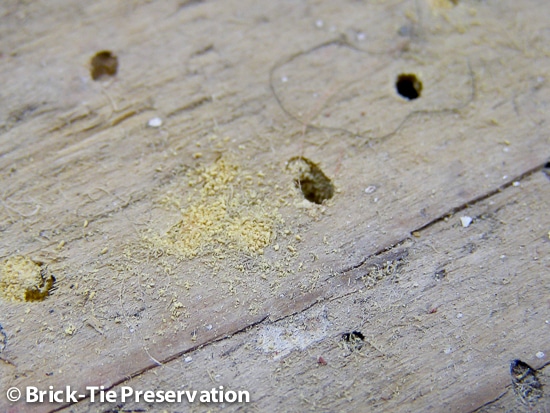The image is a horizontal, rectangular photograph of an old, weathered wooden surface that could be a deck or tabletop. The wood is marked by several holes, cracks, and stains, giving it a rustic and aged appearance. Scattered across the surface are various small items, which might be burs, rocks, or fragments of wood, along with patches of yellow, powdery material that could be sawdust. Additionally, there appears to be bird droppings on the wood. In the lower left corner, there is white text that reads "Brick Tie Preservation," possibly indicating a company name, accompanied by a small circular logo to the right of the text. The image is brightly lit and very clear, showcasing the intricate details of the wood grain and the assorted debris.